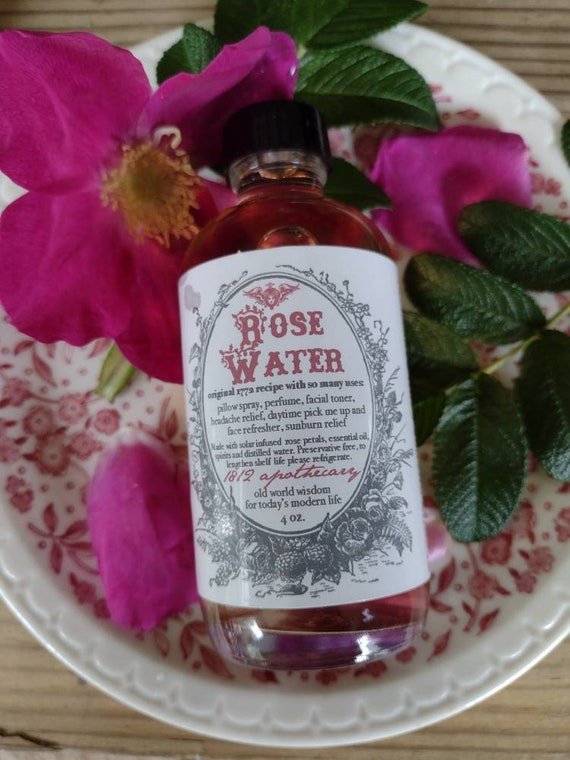The image depicts a bottle labeled "Rose Water" with a black cap, containing a reddish or pink liquid. The white label includes detailed information: "Original 1772 recipe with so many uses - pillow spray, perfume, facial toner, headache relief, daytime pick-me-up, interface refresher, sunburn relief. Made with solar-infused rose petals, essential oil, and distilled water. Preservative-free, lengthen shelf life, please refrigerate. 1812 Apothecary, old-world wisdom for today's modern life." The bottle is placed on a white ceramic plate adorned with magenta-colored flowers featuring yellow centers and green leaves. The setup highlights the bottle and its natural, historical ingredients amidst a visually appealing floral arrangement.